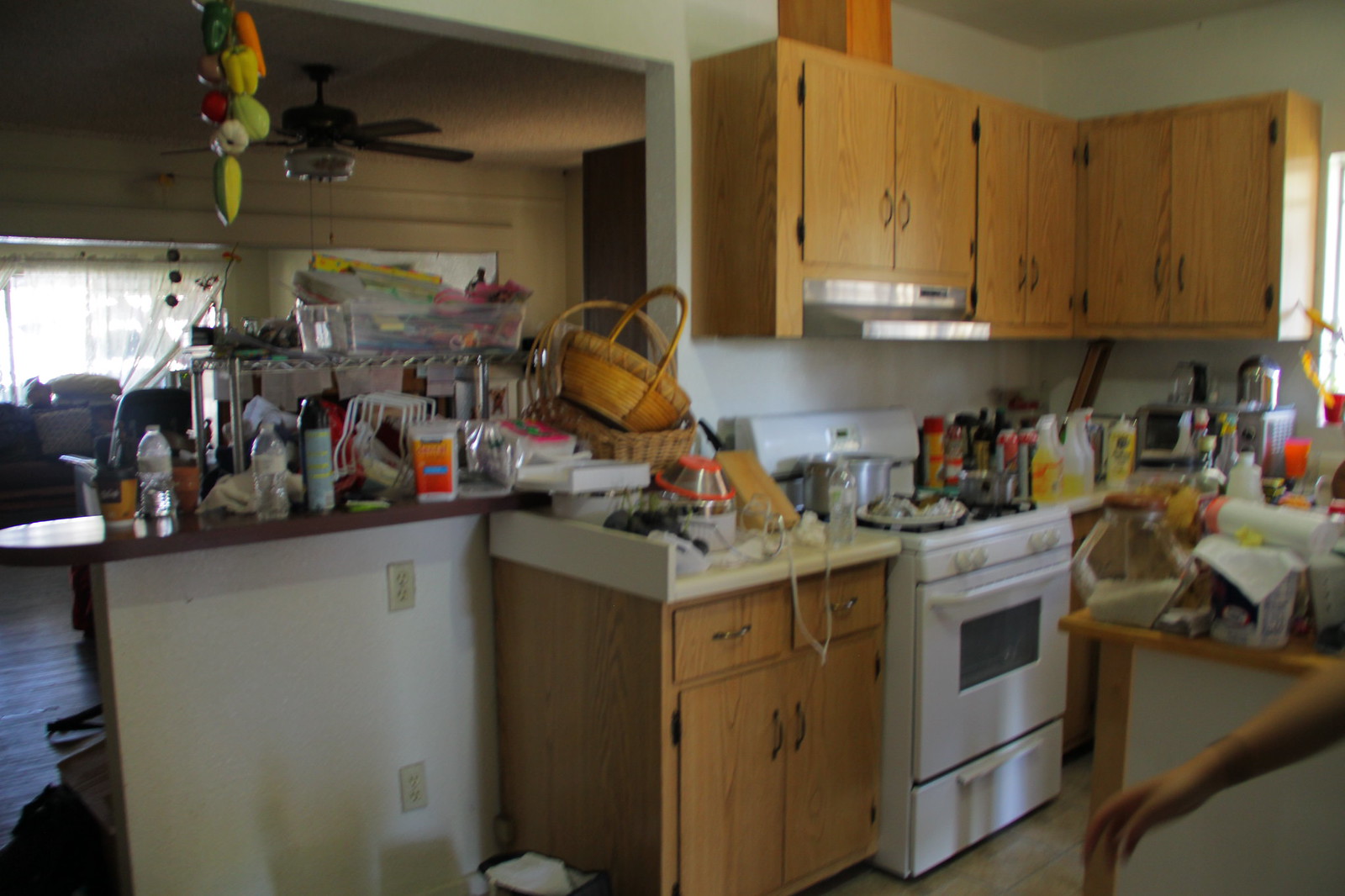This indoor color photograph captures an intimate view of a cluttered kitchen, revealing an abundance of items occupying almost every surface. Starting from the left side of the frame, an opening through the wall offers a glimpse into an adjoining room, which remains obscured due to the clutter adorning the half-wall. This half-wall features a flat island top brimming with various objects, including multiple water bottles, racks, and empty baskets. Notably, the space designed for a refrigerator stands vacant, marked only by the visible electrical outlets on the wall behind.

Adjoining this area, the photograph transitions into a view of the tan countertop, which is equally disorganized with an assortment of items. The dark brown cabinets below add a contrasting element to the scene. As the image moves rightward, the clarity diminishes, but a distinct white oven and range stand out. Atop the range, there's a mishmash of items: a pot and several ambiguous containers scattered across the surface.

Advancing further right, the countertop continues to be a repository for an eclectic mix of cleaning bottles and other nondescript items. Above this countertop, brown cabinets line the wall, while a stainless steel range hood presides over the oven below. The kitchen's background wall, painted a light green, frames an additional section of the L-shaped counter, similarly cluttered.

In the photograph's lower right corner, a person's partially visible right forearm and hand appear. A tattoo encircles their wrist, adding a human element to the scene. The overall lighting of the photograph is ample, though the image remains slightly out of focus, lacking any text or printed words. The entire composition offers a vivid portrayal of a frequently used kitchen space in need of organization.